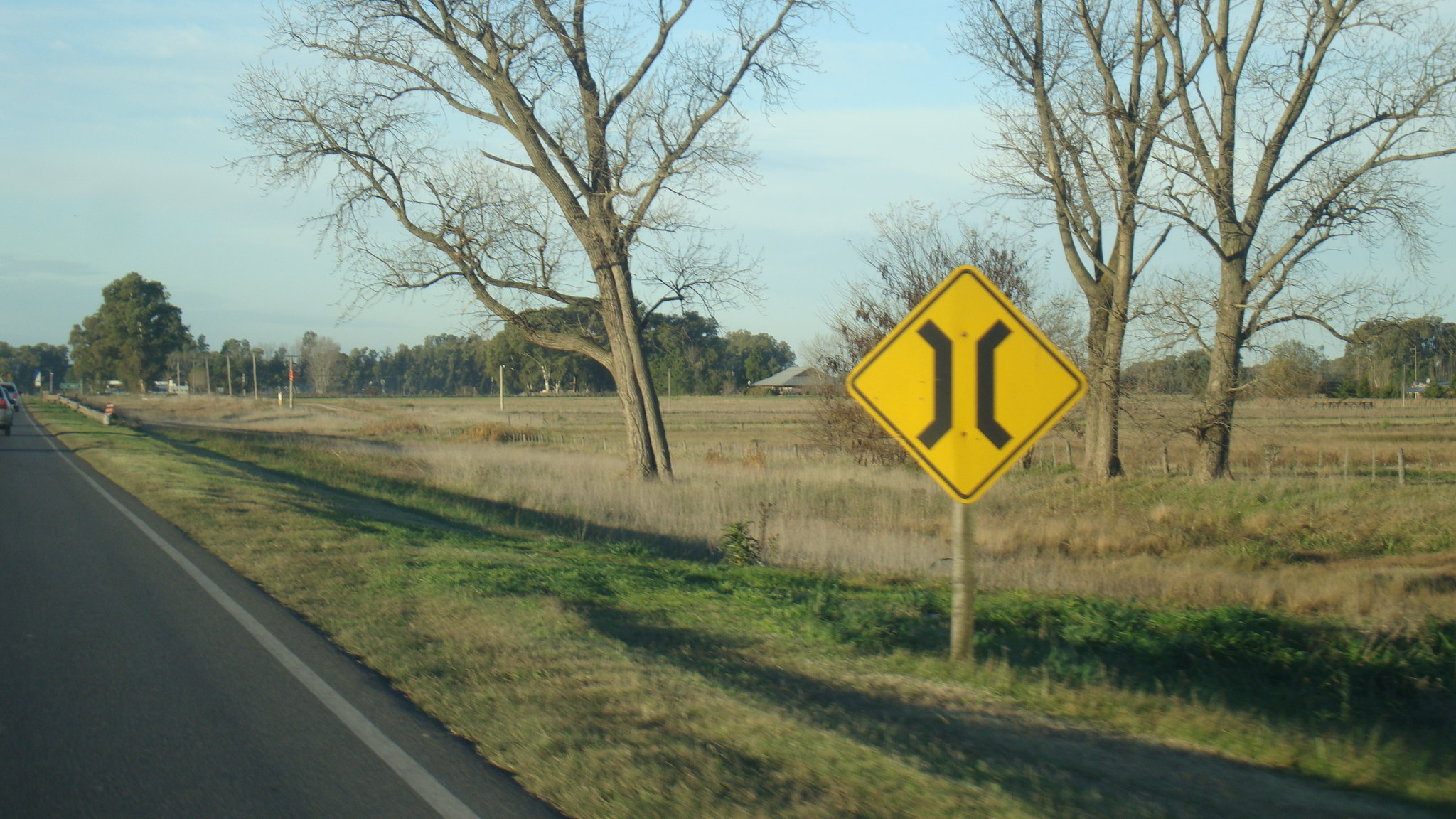The photograph captures a serene rural scene featuring a two-lane roadway bordered by expansive grass fields and dotted with verdant trees. In the bottom left corner of the image, the smooth black pavement of the roadway extends towards the center, where a couple of cars can be seen driving in the distance. The roadway is bordered on its right side by a dark gray line that delineates its edge. 

Flanking the road are fields of lush green grass interspersed with patches of tan, dried vegetation. Several trees, devoid of leaves and displaying brown branches, rise from the grass closer to the middle of the photo. In contrast, the background features a dense array of trees adorned with rich, green foliage. Near the middle of the image, a prominent, diamond-shaped yellow road sign stands tall, marked by two intersecting black geometric lines.

Above it all, the backdrop is a picturesque, light blue sky, indicative of a bright, sunny day, which adds a peaceful ambiance to this rural landscape.